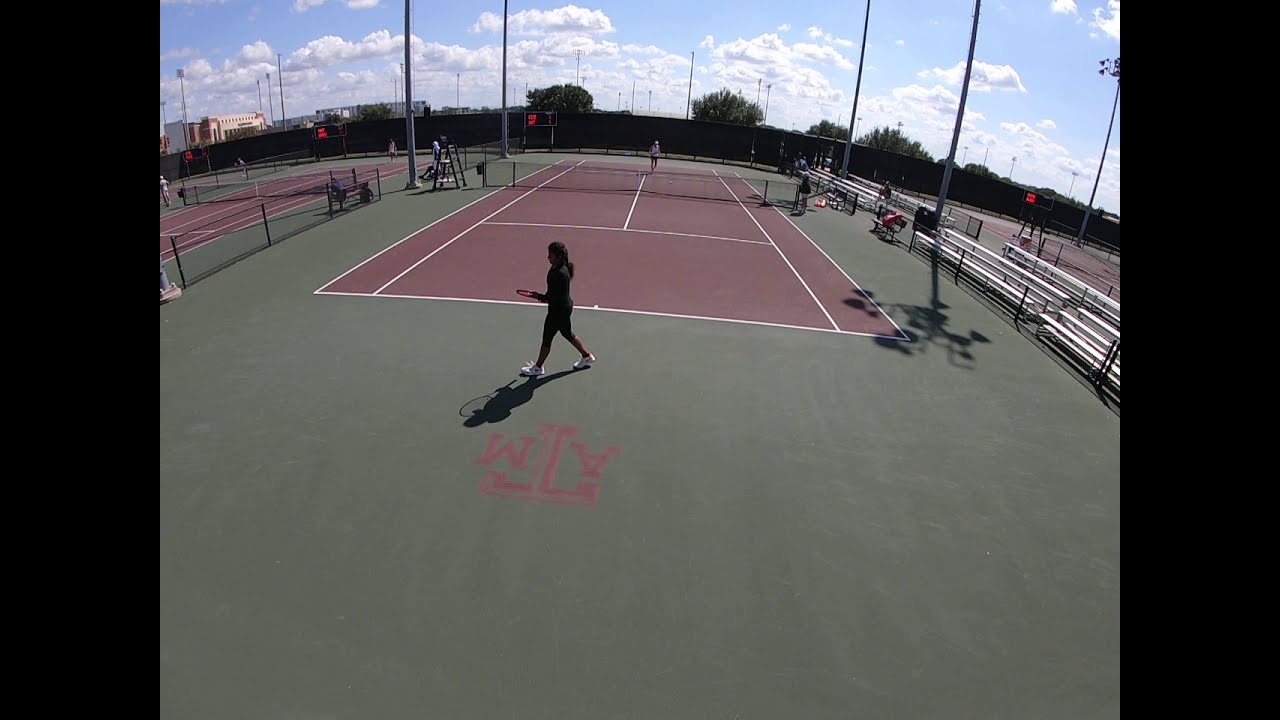In this semi-overhead view of a tennis court complex at Texas A&M, the scene is vibrant with daytime activity. The sky is bright blue, dotted with puffy white clouds, creating a picturesque backdrop. Beyond the dark black fence that encloses the courts, the tops of thick, green trees are visible. The main tennis court in the center features a green base and reddish clay playing surface marked with white lines. On this court, a woman dressed in all-black clothing, including dark shoes, walks towards the left while holding a tennis racket. Another player, indistinct in the far distance on the other side of the net, is also engaged in a game. 

To the right, several empty silver stands are positioned, except for one person whose details are unclear. The initials "TAM" are visible on the ground, confirming the location as Texas A&M. Further to the left, another court is partially visible with some figures in the background, though they remain indistinct. Large poles equipped with lights are mounted around the courts, suggesting provision for nighttime play, though currently unused. The fisheye lens effect slightly curves the edges of the image, adding to the dynamic perspective of this bustling tennis facility.